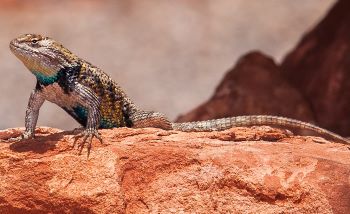In this detailed outdoor photograph taken in a desert environment, we observe a multicolored lizard perched on top of a flat, clay-colored red rock. The lizard, displayed in a side profile from the left, showcases a vivid array of colors: its back features striking yellow scales with black stripes and brown spots, while the underside of its torso is an aqua blue shade blending into white around its neck. The lizard's head is predominantly yellow with a gray mouth region, and a distinctive aqua blue trim runs along the bottom of its chin. The lizard's elongated fingers and two visible limbs rest on the rock, and its long, striped gray tail extends towards the right edge of the image. The background is out of focus but reveals more barren rocks, underscoring the desolate nature of the scene. The photograph captures the lizard in a still, slightly arched position, highlighting its detailed, scaly texture in the bright daytime light, with no other plants, animals, or humans present in the frame.